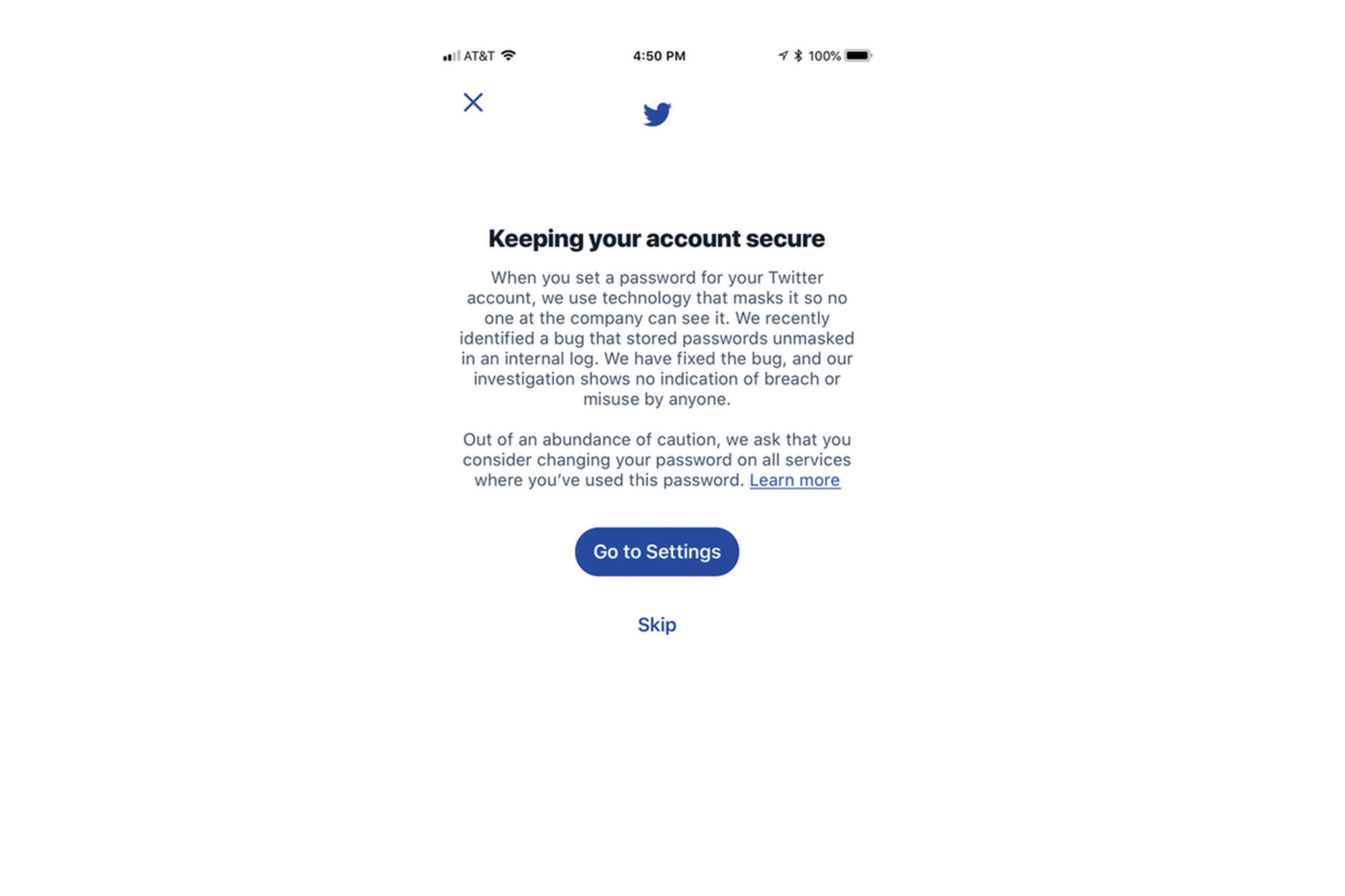This is a detailed screenshot taken from a mobile phone with a white background. In the upper left corner, the screen displays "AT&T" as the network provider, showing two out of five bars of mobile signal strength along with full Wi-Fi connectivity. The time in the center of the status bar reads "4:50 p.m." To the right of the time, there is an indicator showing that location sharing is turned on, a Bluetooth icon, and a battery icon at 100% charge.

Under the status bar, there is a pop-up notification from the Twitter app. In the upper left corner of the pop-up, there is a small blue "X" button. The center of the pop-up features the Twitter icon, a silhouette of a flying bluebird. Below the icon, bold black text reads, "Keeping your account secure." 

The message continues in regular font: "When you set a password for your Twitter account, we use technology that masks it so no one at the company can see it. We recently identified a bug that stored passwords unmasked in an internal log. We have fixed the bug and our investigation shows no indication of breach or misuse by anyone."

Following this, the message advises users: "Out of an abundance of caution, we ask that you consider changing your password on all services where you've used this password." At the end, there is an underlined text in blue, "Learn more," indicating a clickable link for further information.